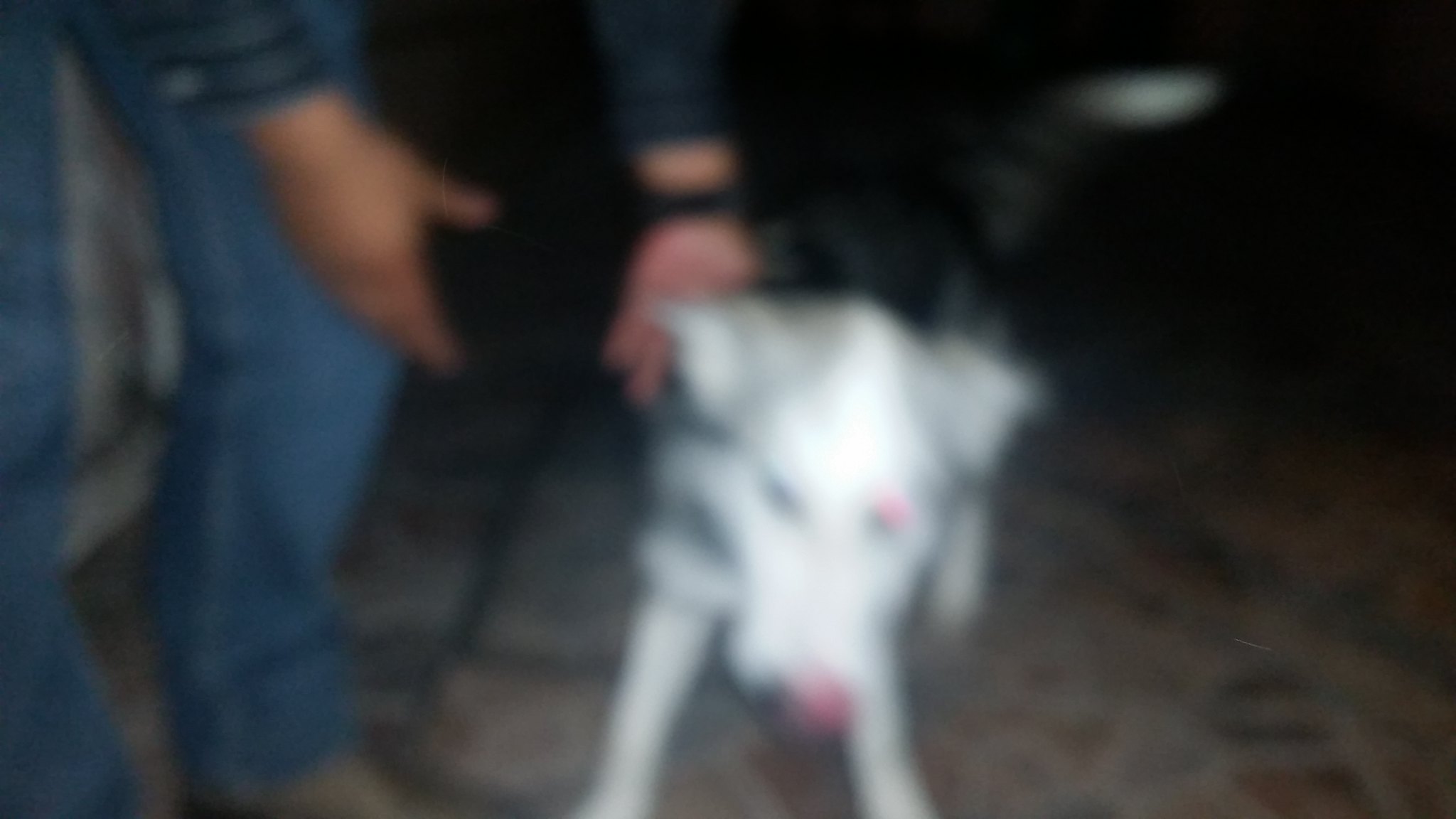In this blurred, out-of-focus color photograph taken at night, the main subjects are a white dog with a pink nose and a pink spot over its left eye, along with a man who appears to be reaching towards the dog. The dog, which also has gray ears and a solid white face, stands on a brown and orange area rug. Its front paws are white, while the back of its body is primarily black, except for the tip of its tail, which is white. The scene seems to be outdoors in a dimly lit area, possibly a cooler environment given the man's attire. The man, dressed in blue jeans, brown boots, and a denim blue jacket, is bent over the dog with his hands open towards it. A wristwatch adorns his left arm, the only part of him visible aside from his legs and hands. The photograph has a dark background, with most details obscured and only hints of the surrounding environment visible.